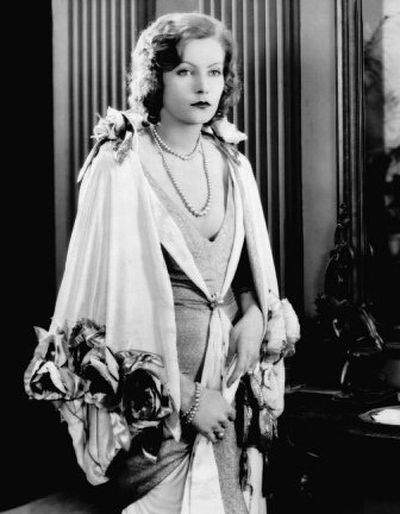This black-and-white photograph, likely from the 1920s or 30s, features the iconic actress Greta Garbo. The image, in portrait orientation, shows Garbo from head to mid-thigh, set against a background of vertical blinds or curtains in a light gray hue. The backdrop includes elements of a movie set with walls, pillars, and furniture vaguely discernible.

Garbo stands at the center of the frame, presenting a serene expression, almost devoid of a smile. She has short, wavy, medium-length brown hair and is adorned with a double strand of pearls draped elegantly around her neck. Her attire is a glamorous, vintage gown with a deep, plunging neckline that reveals her cleavage. The gown, which extends into a long, flowing skirt, features a crisscross pattern and is gathered at the waist. The ensemble includes a cape or shawl attached at the shoulders, embellished with decorative details, and sheer, ruffled long sleeves. 

Her hands, visible and resting gracefully across her hips, reveal a bracelet and a ring on her left hand. The photograph is a quintessential example of vintage black-and-white realism, capturing the elegance and allure of one of cinema's great actresses in a timeless, classic pose.